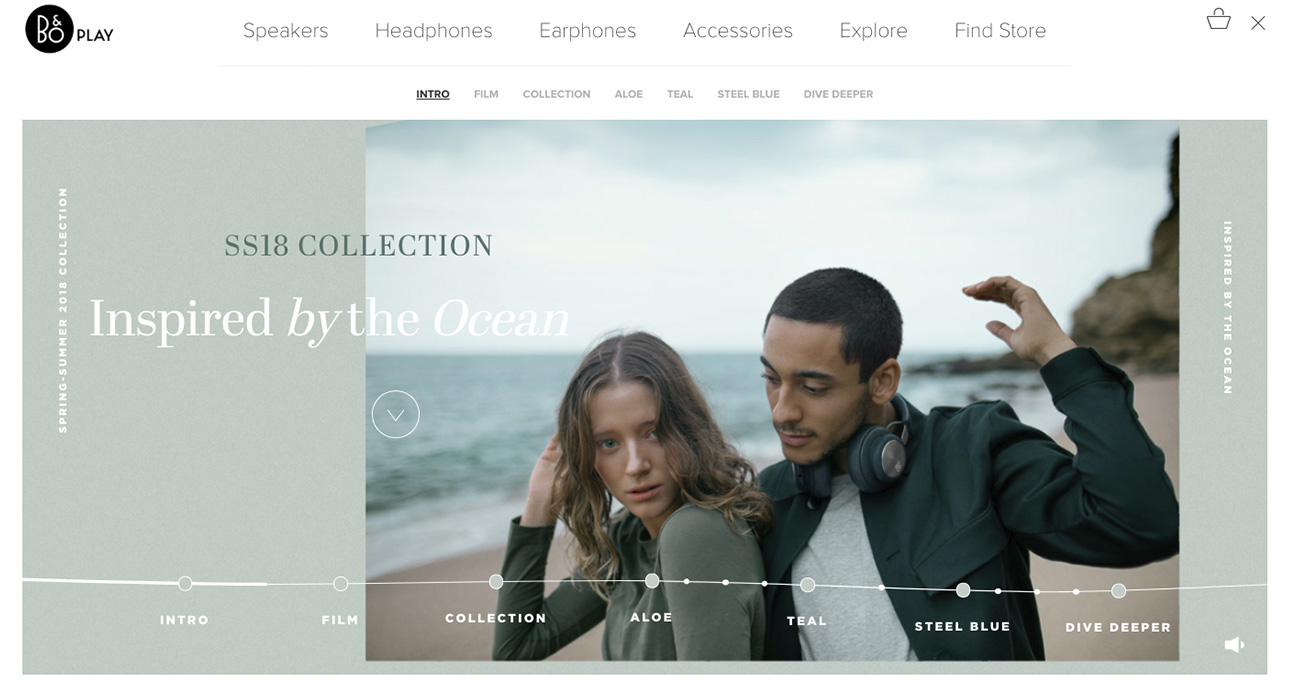This image, in landscape mode, is a screenshot likely captured from a laptop. The interface features a predominantly white background, transitioning to an olive-green background in the second section. 

In the upper left-hand corner, the first row extending across the screen displays several menu options: "B.O. or B.N.O. play," "Speakers," "Headphones," "Earphones," "Accessories," "Explore," "Find," and "Store." On the upper right-hand corner, there is a shopping basket icon accompanied by an 'X' symbol. A thin, centered gray line separates these from the content below.

The active tab is labeled "Intro," marked in black, bold, and underlined text. Other available tabs include "Film," "Collection," "Aloe," "Teal," "Steel Blue," and "Dive Deeper." 

Dominating the lower section of the page is an olive-green background highlighting an image. The image features a light-skinned female dressed in a long-sleeved shirt with seemingly wet hair, and a darker-skinned male wearing headphones, inexplicably positioned in the middle of a beach. He is dressed in a gray shirt and possibly a black jacket. 

On the left side of the image, text reads "Spring/Summer 2018 Collection" followed by "SS18 Collection" in a dark green font, accompanied by the tagline "Inspired by the ocean." A decorative, somewhat whimsical string is situated across the bottom right of the image.

Repeating tabs "Intro," "Film," "Collection," "Aloe," "Teal," "Steel Blue," and "Dive Deeper" are again visible, along with an option to turn off the sound in the bottom right-hand corner.